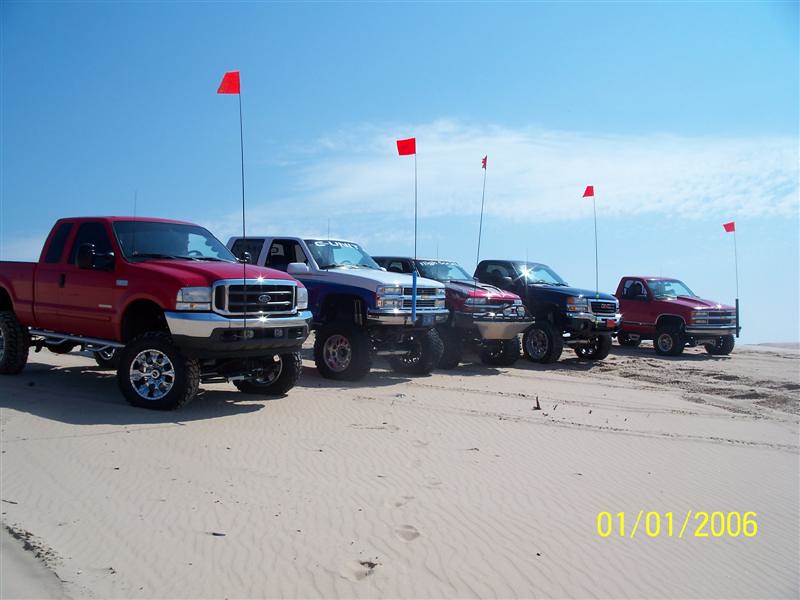This daytime photograph, taken on January 1st, 2006, captures a lineup of five elevated trucks positioned side by side on a sandy desert terrain under a bright, baby blue sky adorned with wispy cirrus clouds. Each truck is equipped with a tall, approximately 20-foot pole mounted on its front bumper, topped with a bright red flag waving in the air. The trucks are identified as a Ford, two GMCs, and a pair of trucks branded "Chubby." Sunlight glints off the windshield of one of the trucks, and there are no drivers visible within any of the vehicles. The scene is accented by a yellow date stamp in the lower right corner, marking the start of the new year.